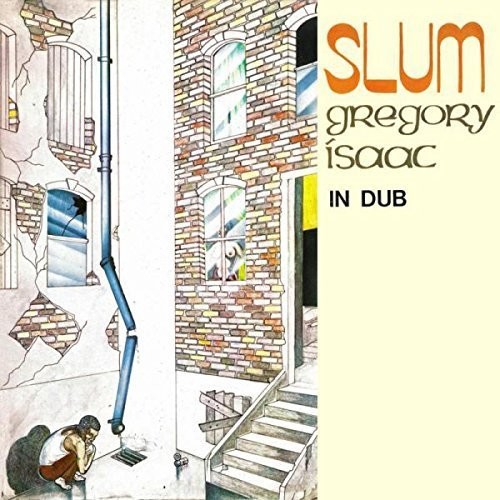The image is an album cover featuring an illustration divided into two distinct sections. On the right side, occupying about one-third of the width of the image, is an eggshell-colored vertical strip. At the top of this strip, in curvy orange text, reads "SLUM," followed by "Gregory Isaac" in greenish-gray text, and "In Dub" in black text below it. These texts are confined to the upper half of the strip. 

The left two-thirds of the image showcases an urban scene illustrated in rich detail. Dominating this area is a dilapidated multi-story brick building with numerous vertical rectangular windows, some of which have arched tops. Through one window, a nude woman is visible, while another window is boarded up, and a third has significant damage with a hole and cracks. The building's plaster is crumbling, revealing the bricks underneath.

The left side features a metallic downspout leading to a gutter on the street. Near this gutter, huddled against the wall, is a black man with short hair. He is wearing a white tank top and red pants, barefoot, and appears to be in a crouched, vulnerable position, with his shadow cast on the wall behind him.

A stone staircase on the right side of the building ascends to an open doorway, contributing to the scene's sense of decay and neglect. The image employs a color palette of yellow, orange, gray, black, various shades of red and brown, maroon, and blue, enhancing the gritty atmosphere of the urban environment.